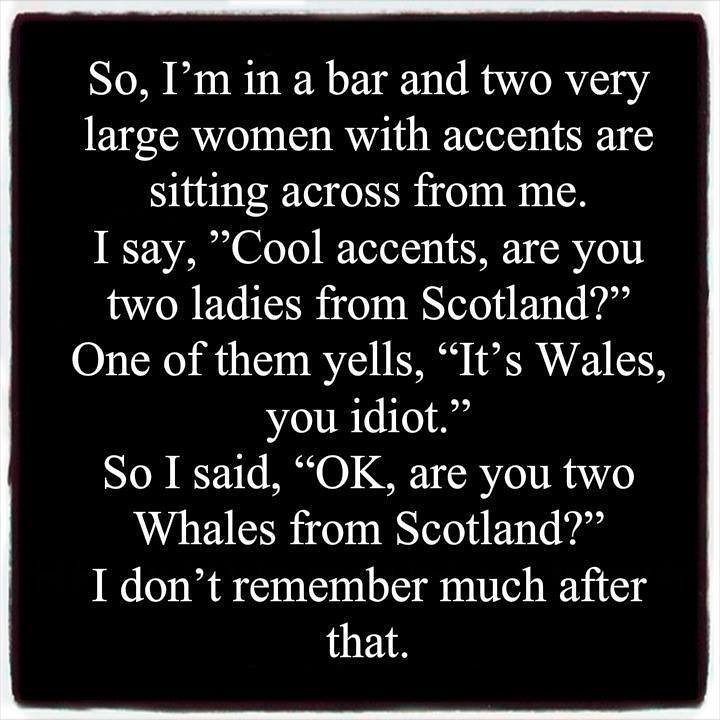**Caption:**

In a stark and minimalist black background, a block of white text is framed by a thin white border, occupying a significant portion of the square image. The text, rendered in a plain, unadorned font, tells a crude and immature joke. The narrative recounts a man's encounter with two large women at a bar, characterized by their distinctive accents. Mistaking their origins, he asks if they are from Scotland. One woman corrects him angrily, stating, "It's Wales, you idiot." Misunderstanding, he then inappropriately asks if they are "whales from Scotland," leading to an implied, unfortunate outcome that he cannot clearly remember. The simplistic, monochrome color scheme underscores the coarse humor of the text, casting an arguably tactless and juvenile tone over the entire image.